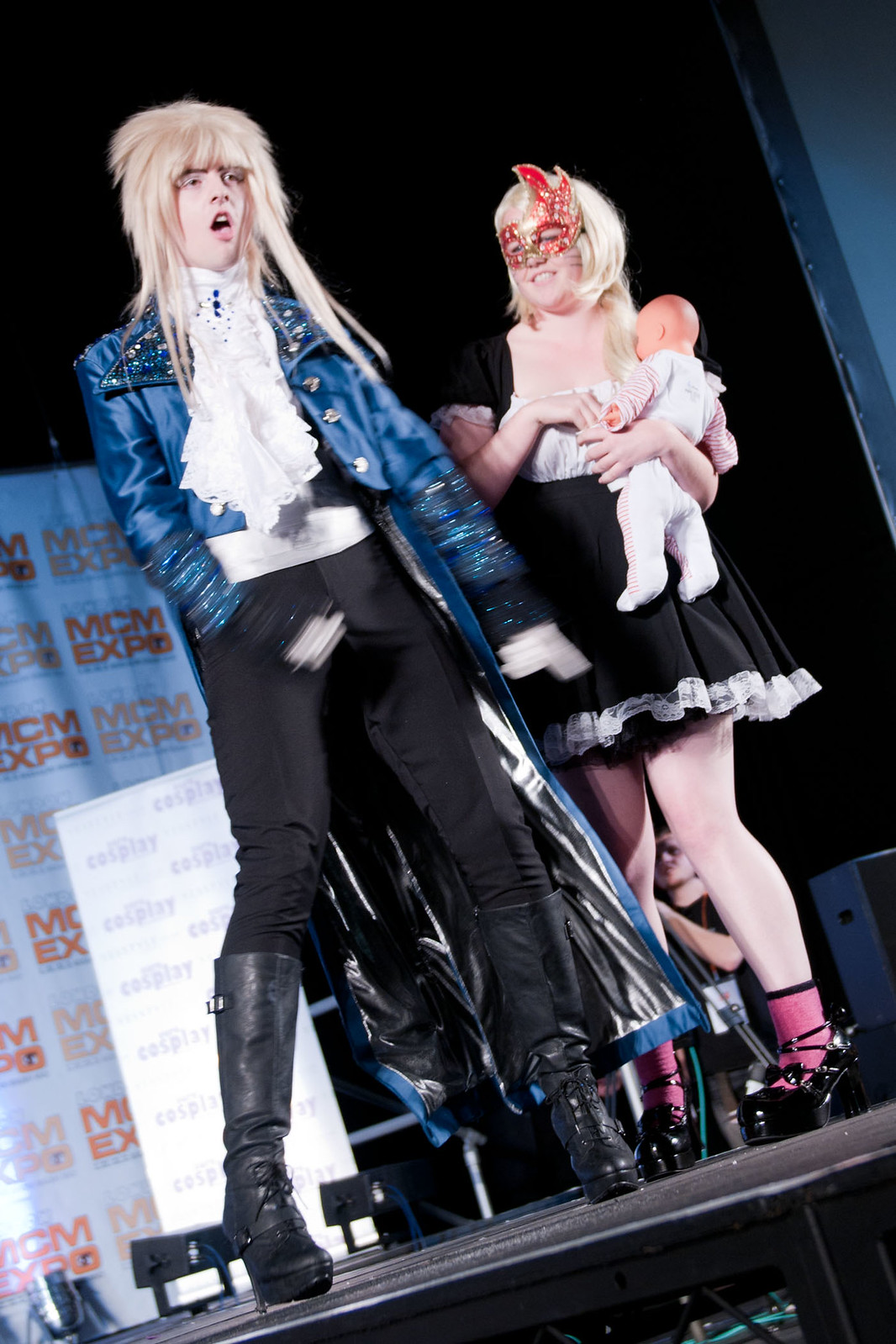In this image, a man and a woman are performing on stage at what appears to be an MCM Expo, with a backdrop prominently displaying the expo's logo and the word "cosplay." The man is dressed in a striking ensemble reminiscent of the Rocky Horror Picture Show. He wears black heeled boots, tight black pants, a flowing white shirt with ruffles, and a vibrant blue leather jacket. He also sports a blonde wig similar to David Bowie's iconic style. To his right stands a woman in a black maid dress with white frills, black high heels, and pink socks. She has a red mask covering her eyes and is holding a baby doll. Both characters seem to be deeply engaged in their performance, creating an intriguing, cosplay-inspired tableau.